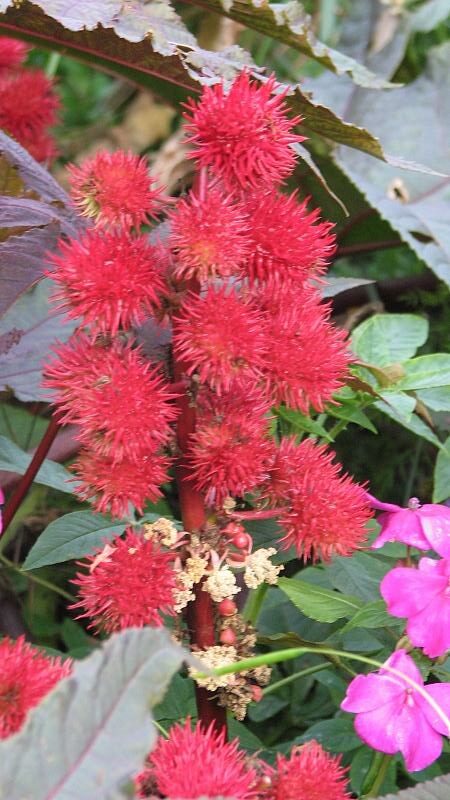The image showcases a unique and vivid plant set outdoors. The central focus is a red stalk adorned with approximately 14-15 striking red spiky ball flowers, reminiscent of koosh balls or pom poms. These red floral spheres, despite their spiky appearance, seem like they might be soft to the touch. The background features a lush tapestry of green leaves, accented by leaves with purplish tones to the left. The bottom right corner reveals several five-petaled flowers in a purplish-red hue. Further down the red stalk, clusters of white flowers and unbloomed red buds are visible, adding to the intricate and captivating composition of the scene.